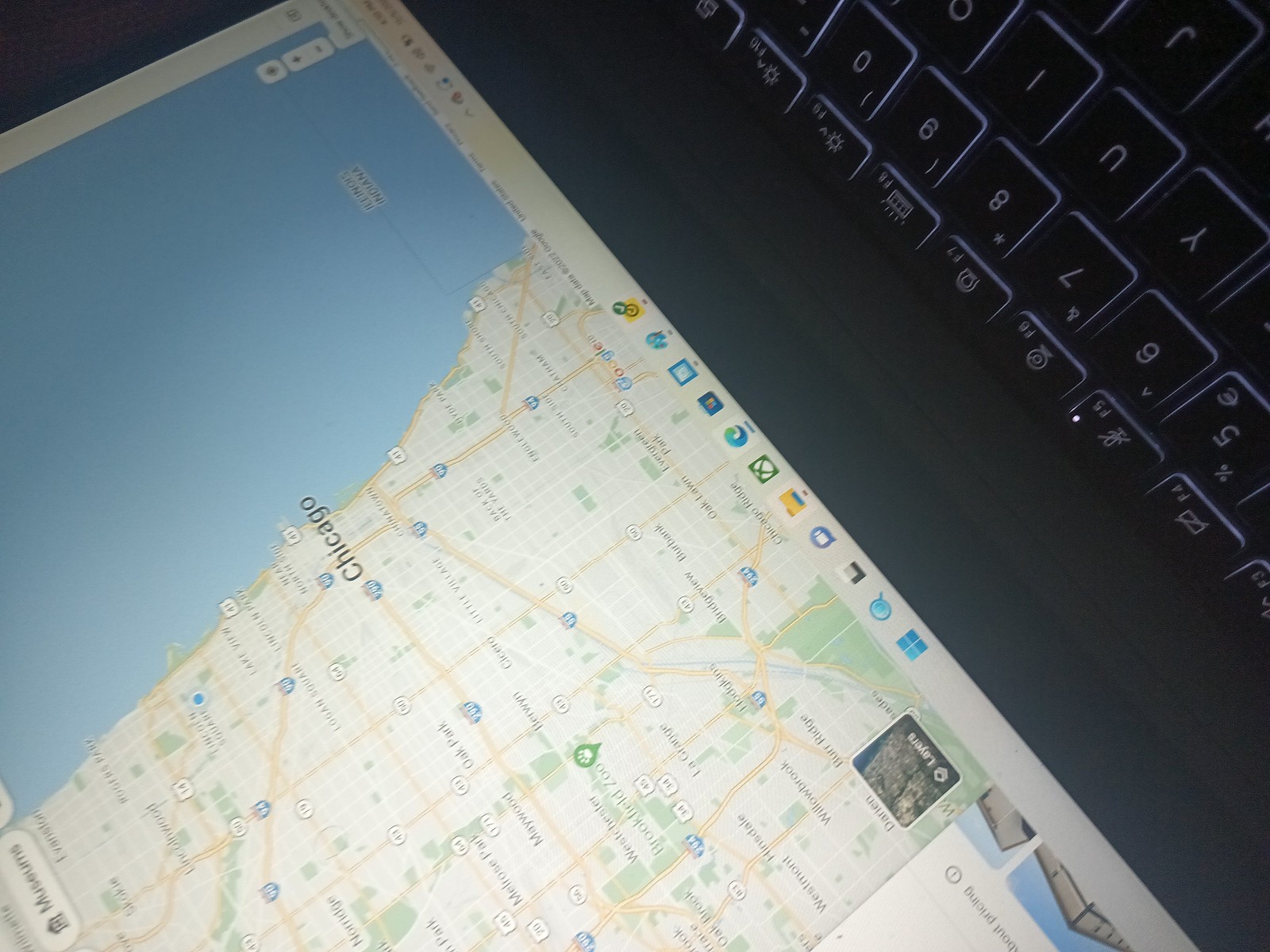This is a color photograph showcasing a laptop viewed from an unconventional, seemingly upside down, perspective. The black keyboard features white backlighting around the edges and clearly visible white letters and numbers, concentrated towards the upper right-hand corner of the image. In the upper left-hand corner, a dark, nearly black triangle is discernible. The partially visible laptop screen is also oriented upside down, displaying a map with a grid overlay. The map prominently features Chicago and covers various regions with white as the primary background color, intersected by yellow grid lines and punctuated by green areas. A bar of icons runs horizontally across the middle of the screen, hinting that the laptop operates on a Windows platform. Additional icons are located towards the right-hand side of the screen. At the bottom left of the map, a small logo is present, alongside another white logo with picture elements, suggesting the use of Google Maps. The map extends to depict a section of the sea on the right-hand side.